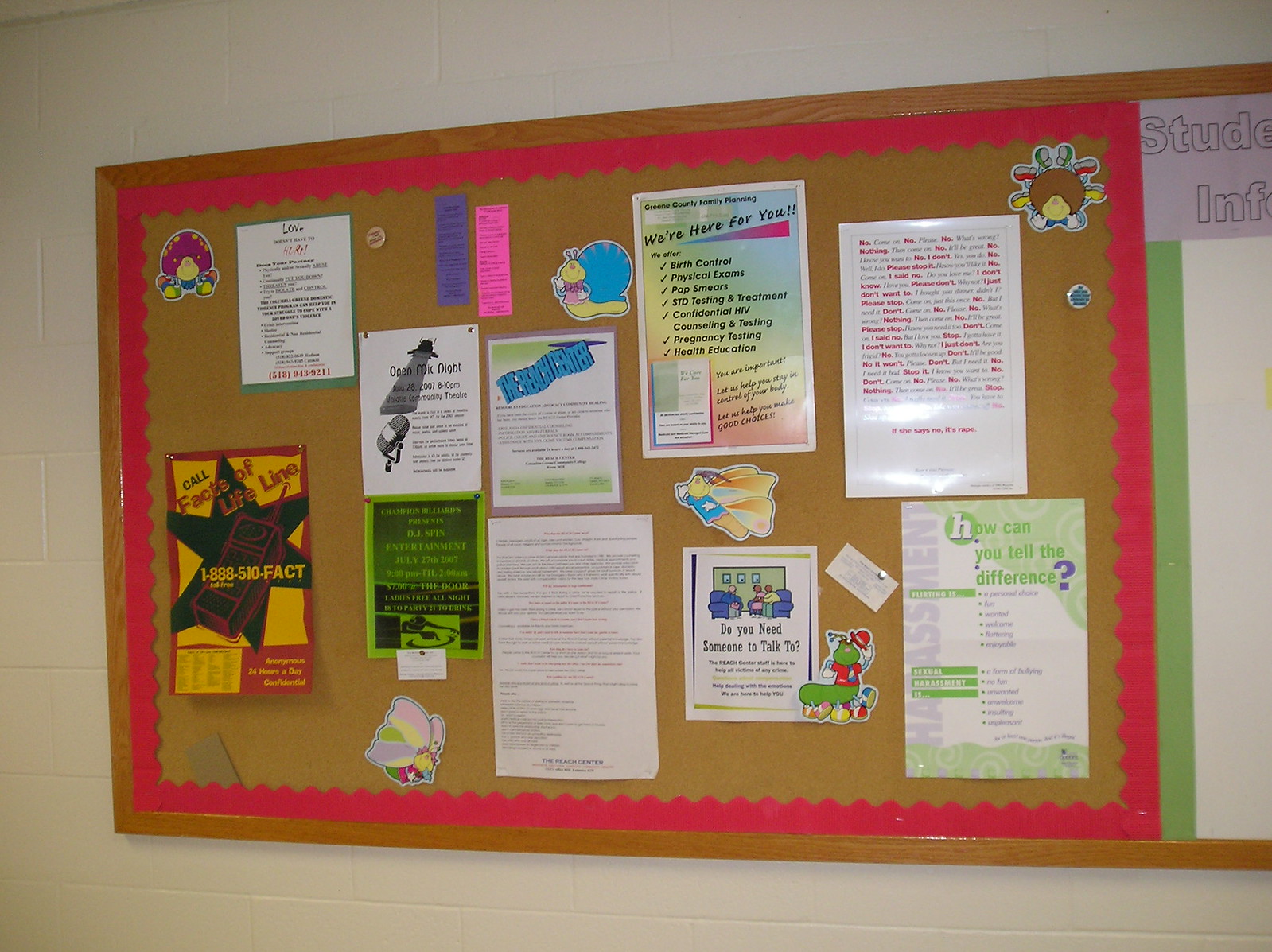This photograph, likely taken in a school setting, depicts a large cork bulletin board mounted on a white-painted concrete block wall. The bulletin board, encased within a wooden frame, features a distinctive red wavy banner that trims its edge. The background of the board is a brown pegboard texture, and it is adorned with numerous posters and flyers of varying sizes and colors that announce different events and information.

Notable among the decorations are anthropomorphized bug stickers: a snail donning a t-shirt, a flying figure with dual capes sporting a blue shirt with a white star, a turkey wearing boots, and ladybugs. Flyers are prominently visible, including a multi-colored one near the top right and a green and purple flyer asking, "how can you tell the difference?" Pertinent messages on other flyers read “facts of lifeline” and “we’re here for you,” although some smaller texts are illegible from a distance.

To the left of the cork board, partially visible, is another whiteboard with a green rim. This whiteboard contains a poorly printed poster that likely spells out "STUDENT INFO" in white letters outlined in black, characterized by the visible characters "S-T-U-D-E" and "I-N-F." Overall, the photograph captures a lively and informative school bulletin board filled with a mishmash of educational and decorative elements.